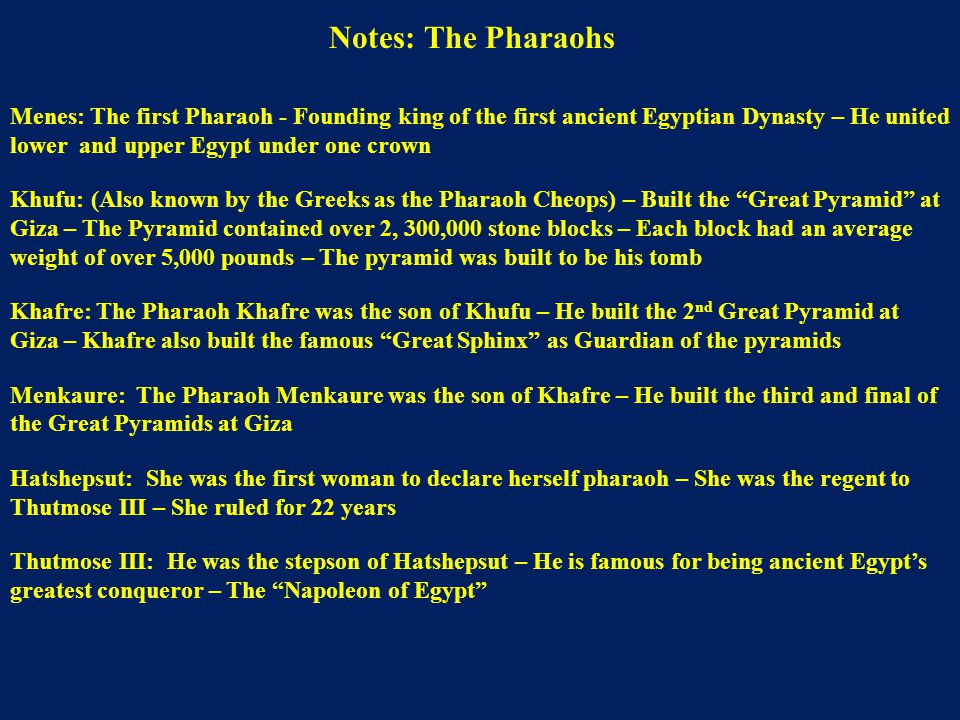The image is a square with a black background that appears blue, filled with yellow text in a typeface resembling Times New Roman. It has the appearance of a PowerPoint slide. The title, "Notes: The Pharaohs," adorns the top, introducing a detailed list of ancient Egyptian pharaohs and their notable achievements. 

Starting with Menes, the first pharaoh and founding king of the first ancient Egyptian dynasty, the text explains how he united Lower and Upper Egypt under one crown. Following Menes, it details Khufu, also known by the Greeks as Pharaoh Cheops, who built the Great Pyramid at Giza. This monumental structure contained over 2,300,000 stone blocks, each averaging over five tons in weight, and was constructed as his tomb. 

Next, the image describes Khafre, Khufu's son, who built the second Great Pyramid at Giza and is credited with commissioning the Great Sphinx to guard the pyramids. Then comes Menkaure, Khafre's son, who built the third and final pyramid at Giza. 

The image also highlights Hatshepsut, the first woman to declare herself pharaoh and regent to Thutmose III. She ruled for 22 years. Finally, it mentions Thutmose III, Hatshepsut's stepson, celebrated as ancient Egypt's greatest conqueror, often referred to as the Napoleon of Egypt.